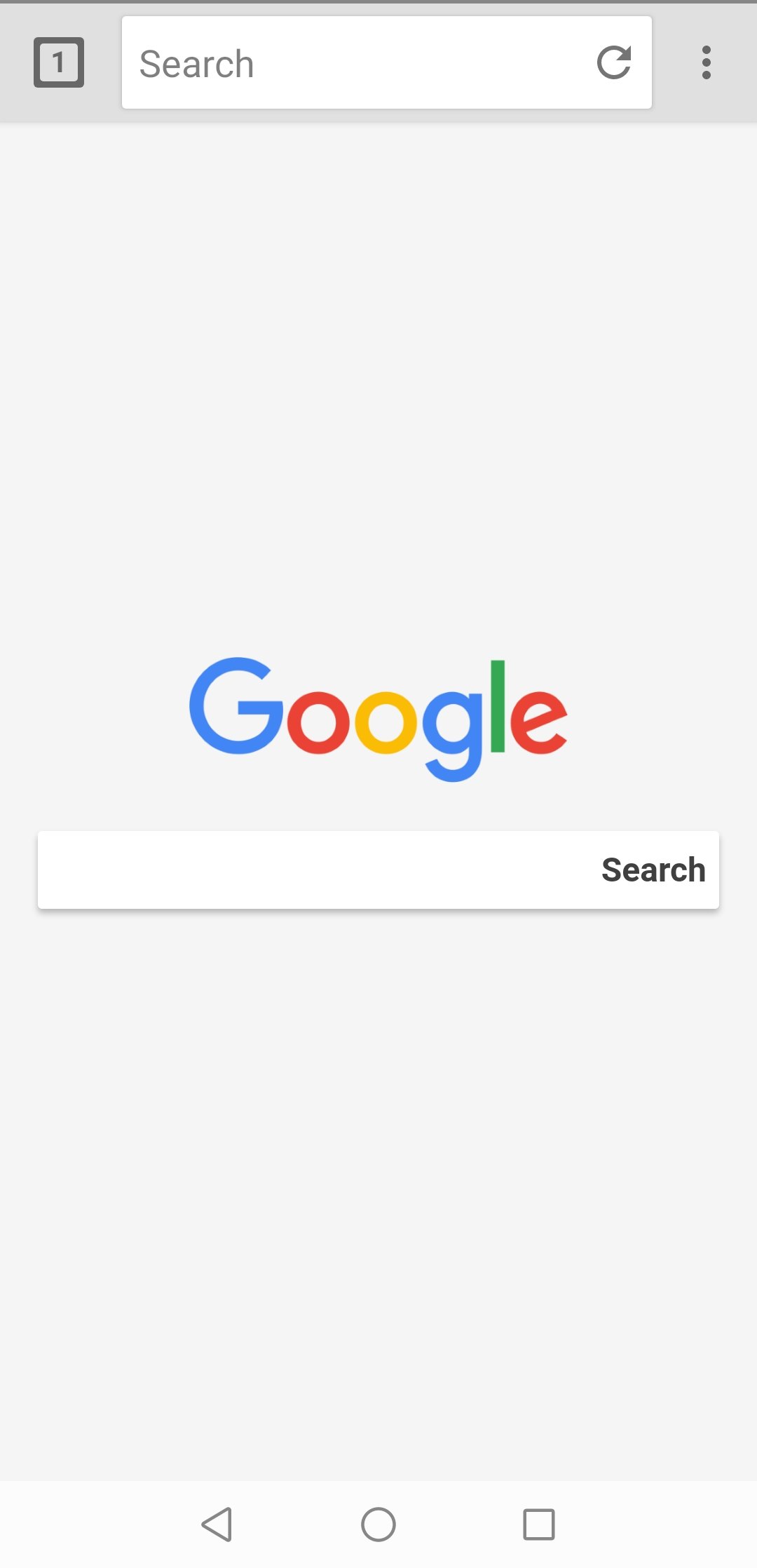The image depicts a smartphone screen displaying a Google search page. The upper part of the screen features a gray navigation bar. Within this gray bar, on the upper left corner, there is a small black square with a white numeral "1" inside it. Adjacent to this, there is a white search bar with the placeholder text "Search" in gray, along with a refresh button next to it. On the opposite end of the gray bar, there are three vertically aligned gray dots, indicating a menu.

Below the gray bar, the main content of the page is displayed against a white background. In the center, the colorful Google logo is prominently featured, with the letters in the following colors: "G" in blue, first "O" in red, second "O" in yellow, "G" in blue, "L" in green, and "E" in red. Underneath the Google logo, there is another white search bar containing the word “Search” in black. The white of this search bar is slightly different from the white background of the page, though both are white.

At the bottom of the screen are navigation icons typical of an Android smartphone: a left-pointing triangle for back, a circle for the home function, and a square for recent apps. These icons incorporate the colors of Google (blue, red, yellow, green) along with gray, white, and black.

Overall, the image suggests the user is viewing a Google search page on a smartphone browser.